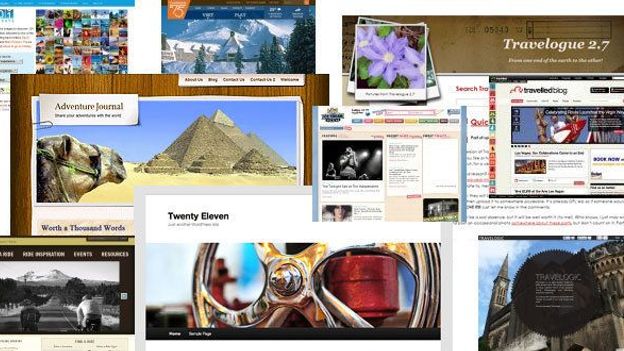This collage showcases an array of travel adventures through a series of captivating images. At the top, there is a vibrant, multicolored picture, setting a vibrant tone for the collage. Just below, a photograph featuring a majestic mountain range paints a serene background scene. In the foreground, an enchanting image captures a camel gazing towards the awe-inspiring pyramids. Beneath this, a striking black-and-white shot features someone standing in the middle of a road with a mountain in the distance, adding a touch of timelessness. Another captivating element is a shiny steering wheel adorned with a red valve, dated 2011, which adds a sense of nostalgia and exploration. Tucked in the corner is a picture of an ancient, grand castle, evoking historical intrigue. Sprinkled throughout are smaller elements, including a delicate purple flower and a diminutive, barely discernible screenshot of another travel moment. The image collectively represents "Travel Log 2.7" from a travel blog, with the adventure themes vividly brought to life through each individual element, creating a rich tapestry of global exploration.